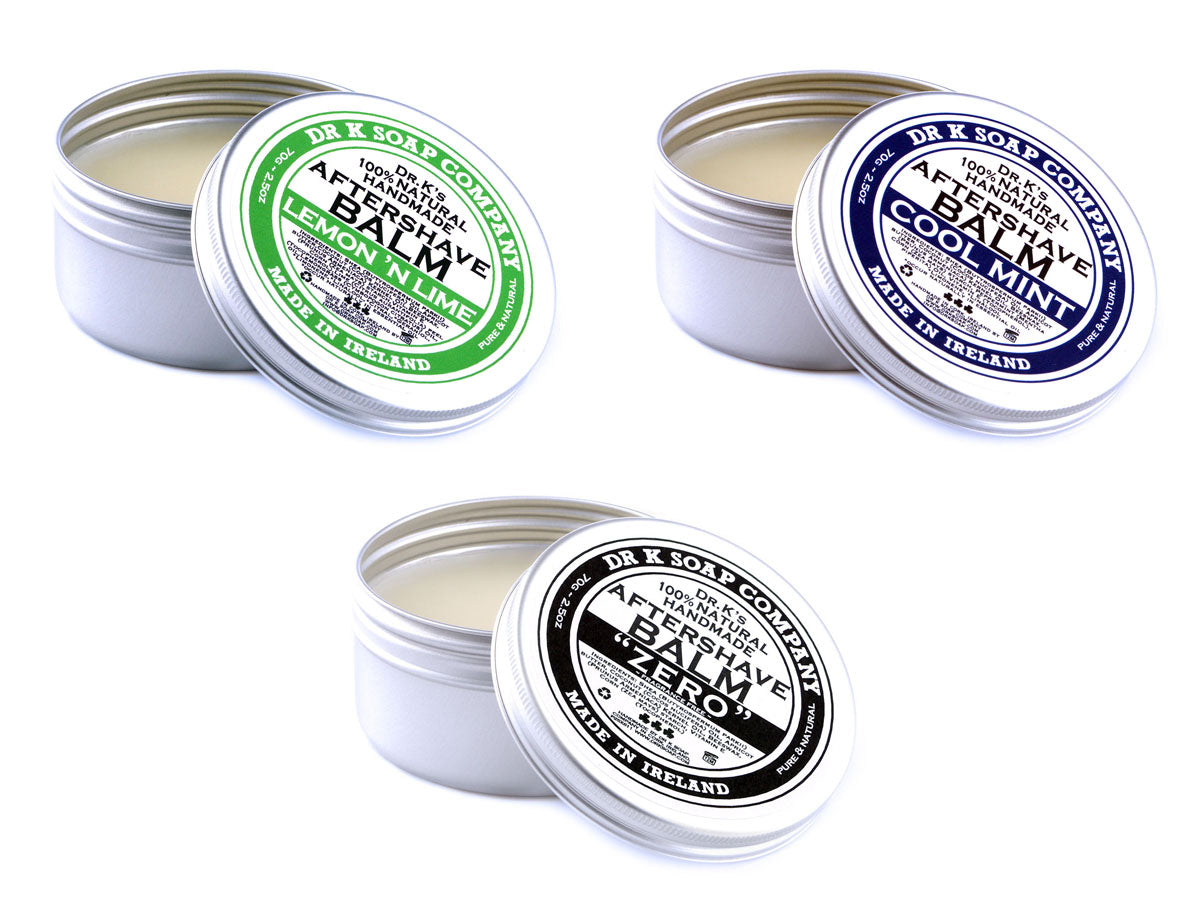This advertisement displays three small, round tins from Dr. K's Soap Company, positioned neatly side by side. Each tin features a classic silver aluminum color around the rims and bottom portion, which is accented by its corresponding color-coded lid. The lids are embossed with the brand's label, "Dr. K's 100% Natural Handmade Aftershave Balm," proudly stating that the products are made in Ireland. 

Inside, the content varies slightly in color, ranging from a creamy off-white to a lighter beige balm. These aftershave balms come in three distinct scents: 

- To the left, the lid with a green ring indicates the Lemon and Lime scent.
- In the center, a navy-blue ring marks the Cool Mint variety.
- Finally, on the right, a lid with a black ring designates the Zero scent, which possibly implies no added fragrance.

The tins are comparable in size to small tobacco containers and hint at a high-quality, natural grooming product designed for post-shaving care.